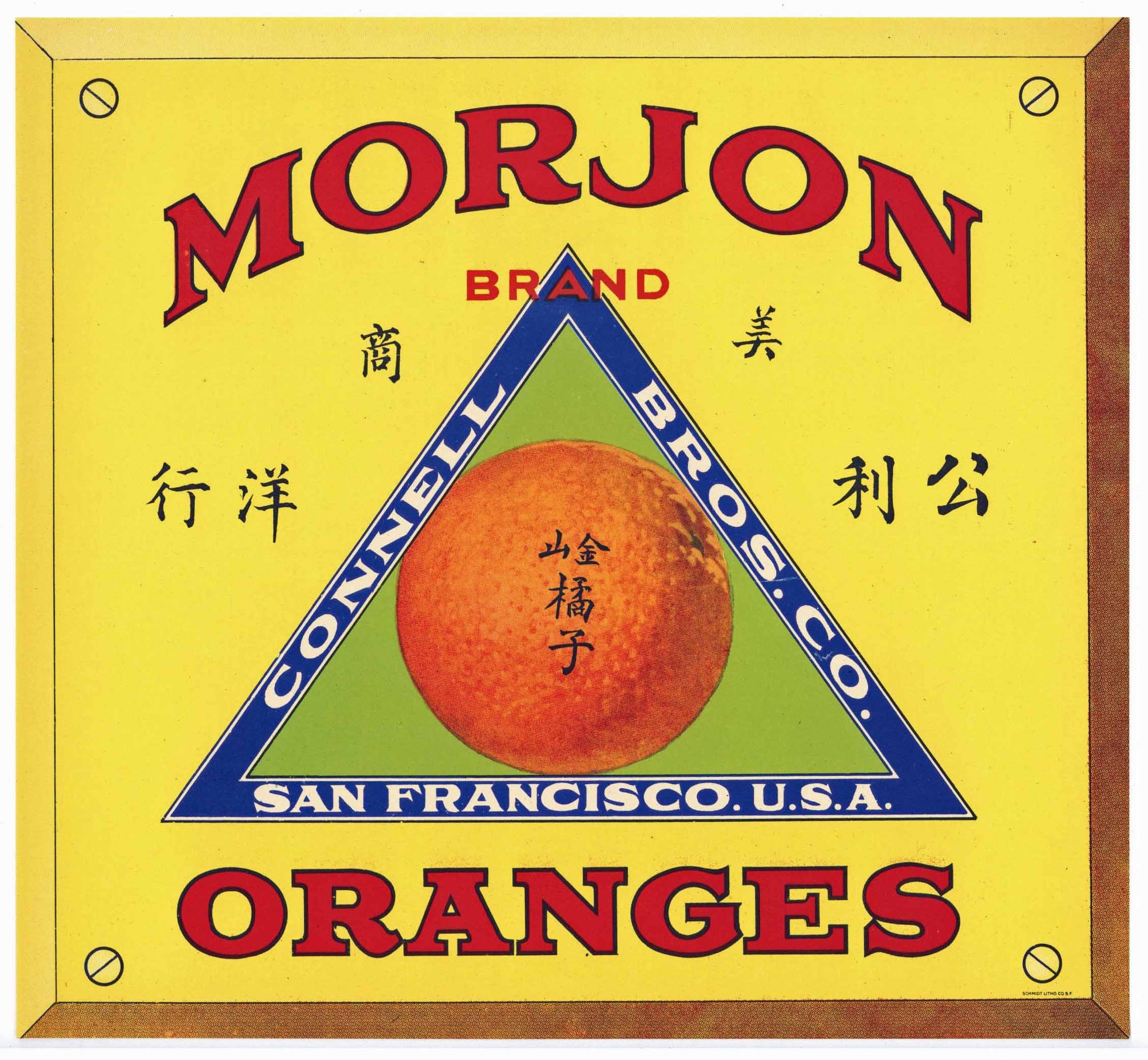The illustration features a detailed logo prominently centered against a white backdrop. At the heart of the image is a yellow square with each corner fastened by screws or rivets, enhancing the design's three-dimensional effect. Inside the square is a bold, red text proclaiming "More John Brand," with "Oranges" written below in the same striking red typeface.

Centrally placed within the square is a blue triangle, and inside this triangle, more information is conveyed. At the triangle's top, crisp white text spells out "Conal Bros. Co.," and directly below, "San Francisco, USA." At the center of the triangle sits an orange, adorned with Asian script, likely kanji characters. Additional Asian characters, presumably Japanese or Mandarin, are positioned on either side of the triangle, framing the entire design.

The placement and combination of these elements, along with the intricate detailing and the linguistic mix, make this logo not just a label, but a visually rich and culturally infused advertisement.